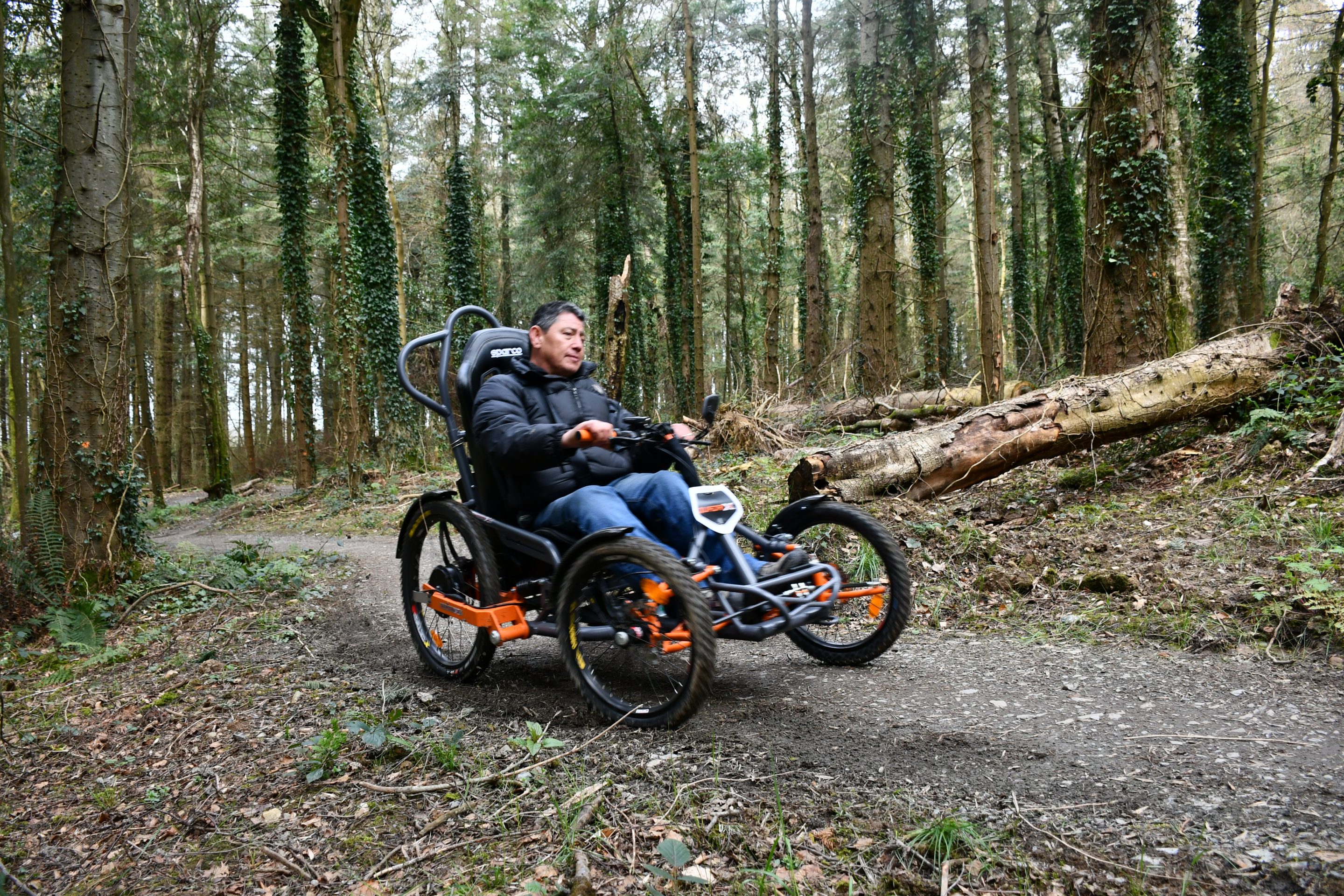The photograph depicts a man navigating through a dense, vine-covered forest on a unique four-wheeled vehicle, which resembles a hybrid between a bicycle and an adaptable off-road wheelchair. Dressed in a large black jacket and blue jeans, the man steers the orange-and-black vehicle, which features spoked wheels akin to those of a bicycle, using handlebars positioned in front of him. The trail beneath him is a dirt and gravel path, flanked by tall trees adorned with vines and leaves, creating a lush and picturesque setting. He is passing by a couple of fallen trees, adding to the rugged atmosphere of the forest. Additional handlebars in a U-shape are visible at the back of the vehicle, suggesting it might also be pushed from behind if necessary. The daylight illuminates the scene, highlighting the natural beauty and serene environment of the woodland path.